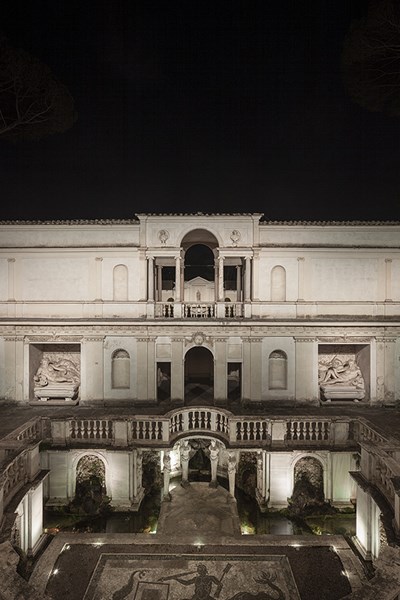This nighttime black and white image showcases a beautifully illuminated historical building, identified as the Etruscan Museum in Rome. The structure is palatial and exudes an air of grandeur. Predominantly white, the museum features a central courtyard, enclosed by lower levels on either side and topped with three stories of balconies and entrances. The intricately designed courtyard boasts arched entryways each adorned with elaborate statues. The central floor is embellished with a detailed mosaic, possibly Roman or Etruscan in origin, depicting a scene with a man wielding primitive weapons. Towering angelic statues and curved columns add to the elegance. Spotlights cast dramatic shadows, enhancing the ornate details and adding depth to the scene. The dark sky behind, with faint silhouettes of trees, frames the museum magnificently.